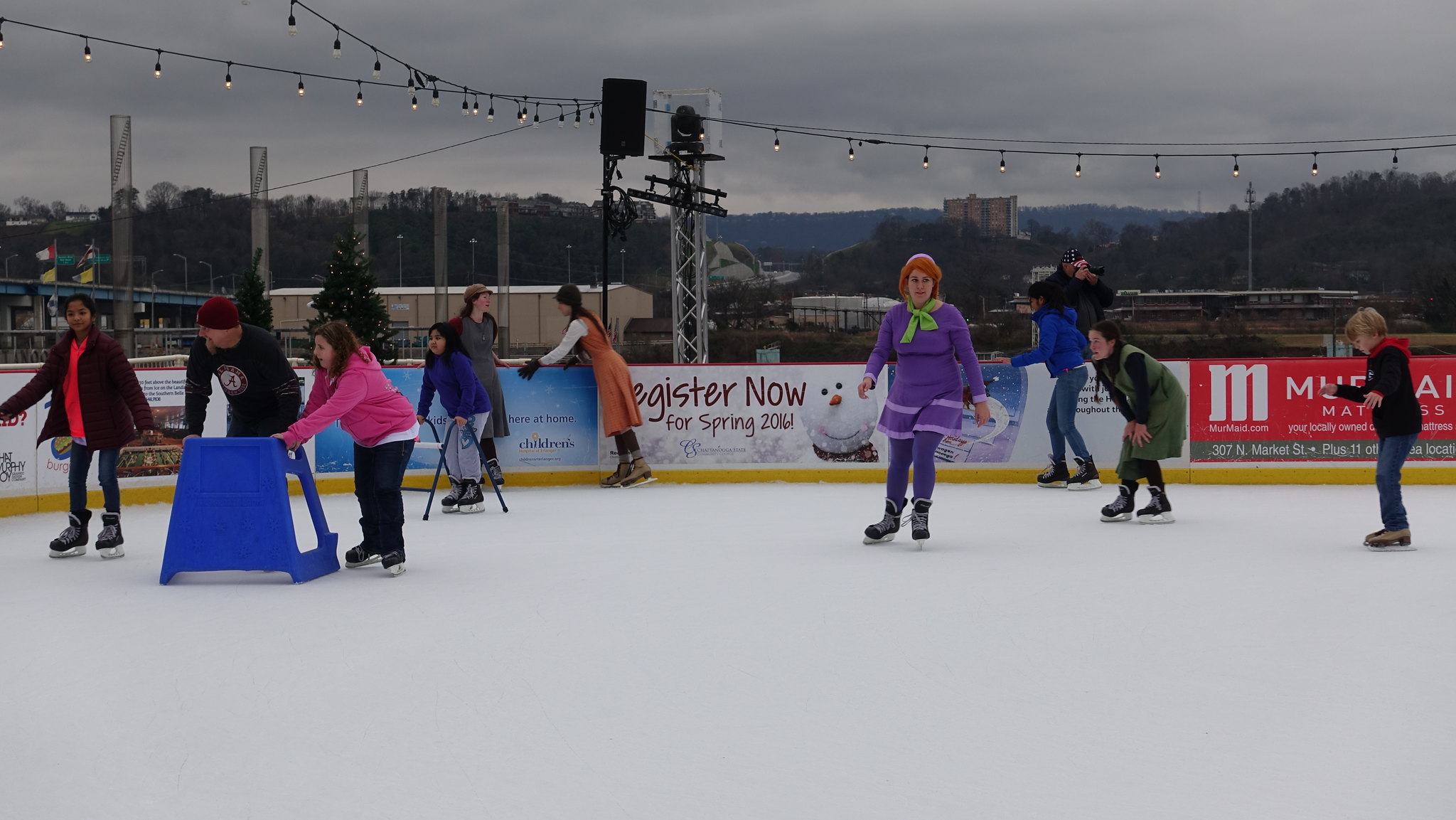The image features an ice skating rink on a cloudy, overcast day, with a gray sky that suggests impending rain or snow. In the far background, hills can be seen, along with a building perched on one of them, adding depth to the scene. Closer, though still distant, are low-rise buildings scattered to the left, center, and right. On the rink itself, there are approximately 10 to 12 skaters, a mix of young to middle-aged individuals, predominantly white with one younger black skater to the left.

The skaters are both children and adults, some using supportive structures like strollers or hand carts to maintain their balance. One notable figure is a woman in a purple dress with a green scarf, which might suggest she's dressed for a special occasion or cosplay. Behind the skaters, a sign on the boards encourages people to "register now for spring 2016," accompanied by a smiling snowman's face. Another man is seen taking pictures, possibly capturing memories of the event.

The image indicates it was taken in the evening, under a band of overhead lights, although it's not completely dark. The rink's edge is lined with banner ads for local businesses, and there's a speaker on a stand likely playing music to enhance the atmosphere. In the background, a tall apartment building and forested areas hint at a small-town setting, completing the cozy and lively scene.